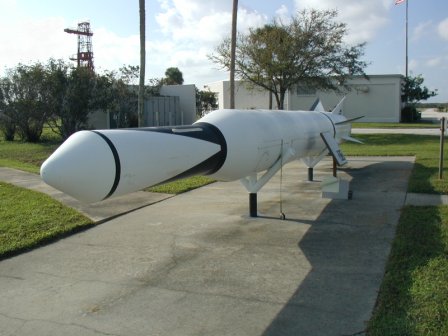The image depicts a white and black missile or rocket on display at what appears to be an outdoor museum, potentially an aerospace or military facility. The missile features green accents around the nozzle, the head, and on its small fins. It is positioned on a slab of concrete, surrounded by well-manicured grass and medium-sized trees. Sidewalks emanate from the pavement, inviting visitors to explore the display. In the background, there are buildings, a tower, and some caged dumpsters. The sky is a clear blue with a few white clouds, suggesting a pleasant, sunny day, possibly during spring or summer. The missile is oriented with its tip pointing somewhat toward the camera, showcasing both its side and front.